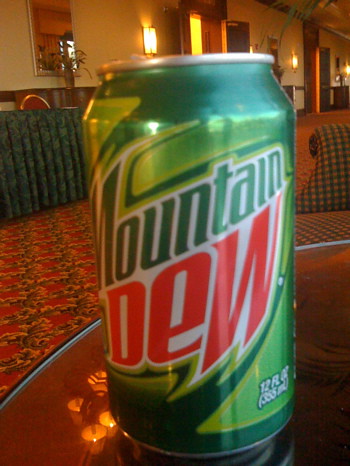This close-up photograph captures a vivid and detailed scene of a Mountain Dew can prominently positioned on a round, shiny brown wooden table. The predominantly green can features the words "Mountain Dew" with "Mountain" in a dark green font and "Dew" in red. The background of the can showcases varying shades of green, from a darker hue to a lime green pattern, with highlights of silver edging at the top and bottom. The front label also indicates it holds 12 fluid ounces, or 353 milliliters. 

The setting appears to be a warm-lit hotel lobby or hallway, with tall ceilings and visible pillars extending into the distant background. Red and brown carpet stretches down the length of the hallway, adorned with several doors and illuminated wall lights. The scene includes decorative elements like a large plant in the upper right corner and artwork in orange and red tones hanging on the walls. Additionally, furniture, possibly a red and black sofa, and other black material furnishing can be seen to the side, adding to the inviting and sophisticated atmosphere of the space. Reflections from overhead lights gleam subtly on the table surface, enhancing the photograph's depth and texture.